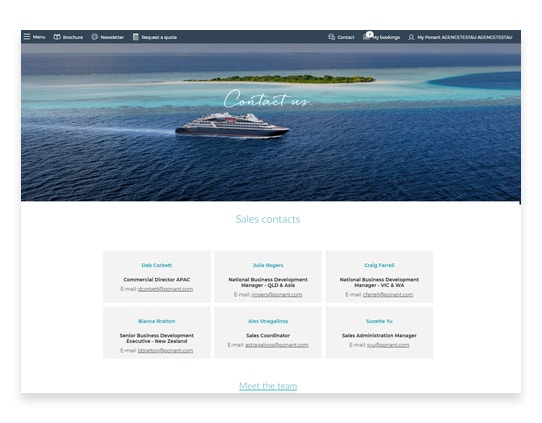The website features a low-resolution design that makes it difficult to discern many details. A dark gray navigation bar with unreadable white text spans the top of the page, although one can vaguely make out the word "menu." Dominating the upper half of the page is an image of a large ocean liner, resembling a cruise ship, set against vibrant blue waters. The phrase "Contact Us" is elegantly written in cursive white letters over the image. In the distance, an island with turquoise waters and lush green vegetation enhances the scenic backdrop.

Below the main image, there is a section labeled "Sales Contacts," featuring names that are difficult to decipher due to the poor image quality. Included in this list are DWB or Deb Carbert, along with names such as Julie, Alex, Monica (or perhaps a name starting with "M"), and Craig. The overall color scheme of the website includes shades of blue, gray, black, white, and green.